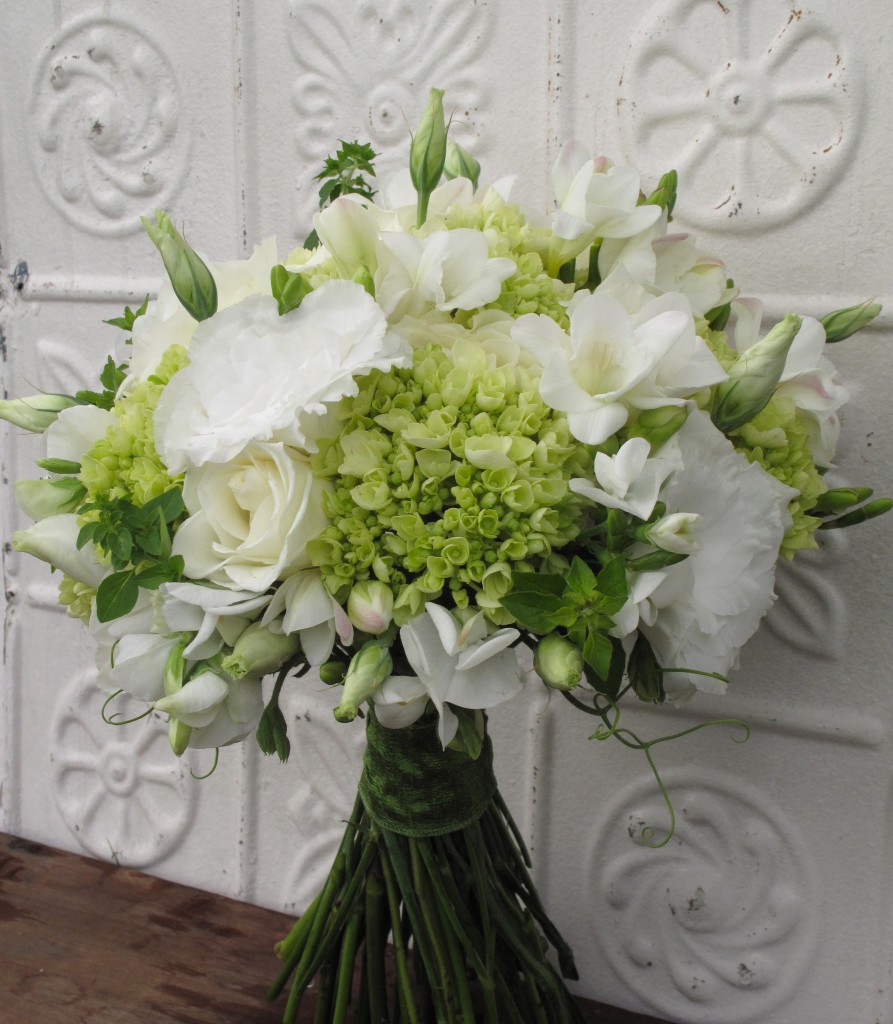The image captures a professionally photographed bouquet of flowers, arranged to possibly be carried by a bride, maid of honor, or bridesmaid at a wedding. The bouquet features an elegant combination of large white flowers, smaller light greenish-whitish flowers, and dainty white blossoms, accentuated by delicate viney stems. The greenery is abundant, with vibrant green stems gathered neatly with a sheer translucent green ribbon. The arrangement exudes a sense of sophistication and beauty.

Resting on a brown wooden surface that has patches of white, the bouquet is set against a fascinating three-dimensional wall of tile. This intricately designed backdrop features an array of patterns, including circular shapes and butterfly motifs, adding depth and artistic flair to the scene. The overall composition, with its rich textures and meticulously crafted floral design, creates an aesthetically pleasing and detailed visual experience.